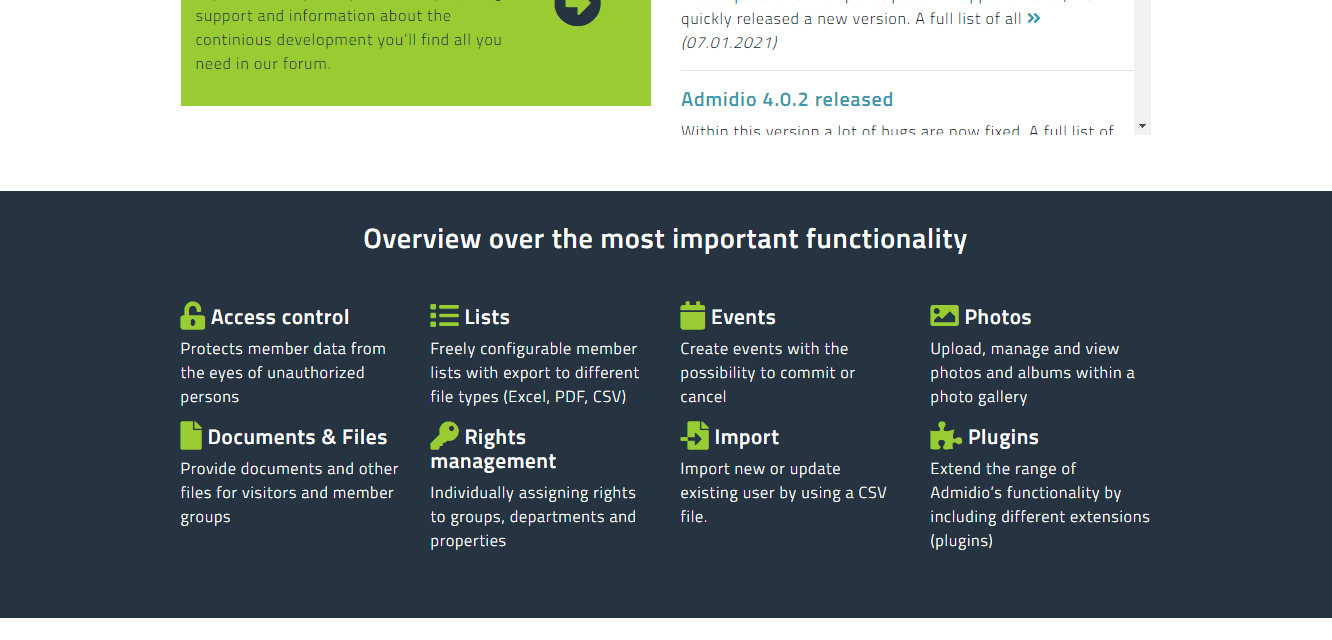This screenshot showcases the bottom half of a web page, divided into two main sections: a white upper section and a navy-blue footer. 

**Upper Section:**
- On the middle left side of the white section, there's a small green rectangle containing the text: "Support and information about continuous development you'll find all needed in our forum." Adjacent to this text is an arrow enclosed in a circle, directing attention towards additional text that resembles patch notes. These patch notes detail various version releases, including notes like "quickly released a new version," though some of the specific text is illegible. One of the visible release dates is 07-01-21.
- Below this, there are additional patch notes for earlier version releases. For instance, there's a note stating "Ad Medio 4.0.2 released," followed by more descriptive text about the update.

**Footer Section:**
- The navy-blue footer features multiple icons and descriptions arranged horizontally in a grid-like pattern. Each entry in this grid includes a title, an icon next to it, and a brief explanation of the feature it represents. This section provides further information about the company or program to which this website belongs.

This structured layout highlights ongoing development updates and company features, effectively guiding the user through the provided information.